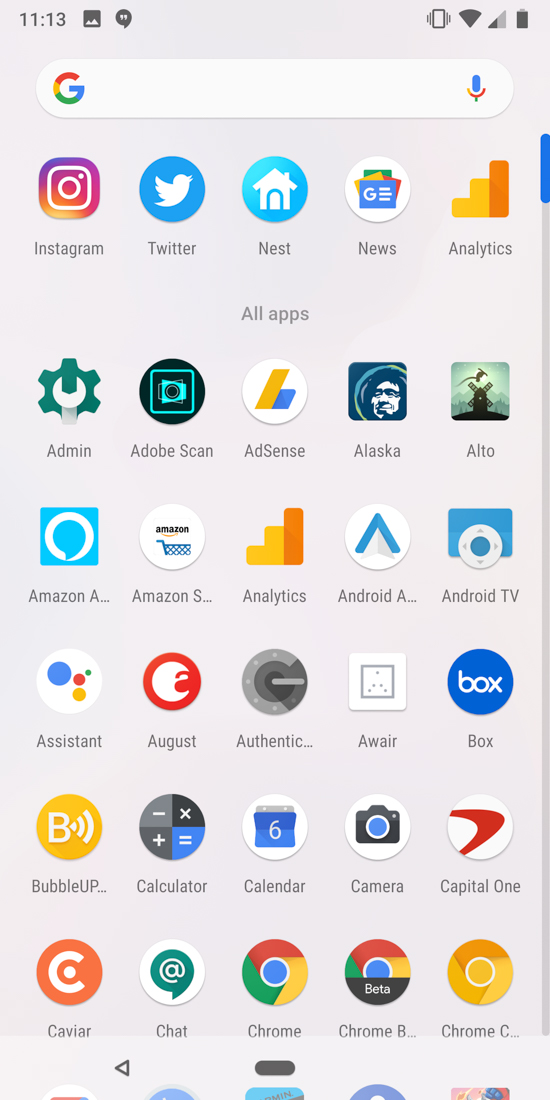Screenshot of a smartphone displaying the app drawer interface. The Google search bar is the topmost element, followed by a horizontally arranged list of suggested apps. Beneath this is the "All Apps" section arranged in a 5x5 grid format.

The apps are displayed in the following order:

**Top Row:** 
1. Admin
2. Adobe Scan
3. AdSense
4. Alaska
5. Alto

**Second Row:** 
1. Nexro
2. Amazon 
3. Amazon Shopping
4. Analytics
5. Android

**Third Row:** 
1. Android TV
2. Assistant
3. August
4. Authentic
5. Aware

**Fourth Row:** 
1. Box
2. Bottle 
3. Up
4. Calculator
5. Calendar

**Bottom Row:** 
1. Camera
2. Capital One
3. Caviar
4. Chat
5. Chrome B
6. Chrome C

The time is displayed at the top right corner showing "11:13," accompanied by the battery icon and the screenshot notification icon.